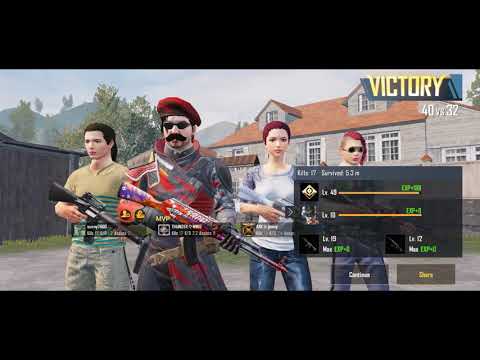The image appears to be a screenshot from a video game, likely a shooter, illustrating a victory screen with the word "Victory" in orange text at the top right, next to the score "40 vs 32" in white letters. The picture is framed with black borders on the top and bottom. In the center, four characters are standing in a line facing forward, each holding rifles. From left to right:

1. A male character with black hair, wearing a yellowish (or green) shirt and gray pants (or green shorts), holding a large gun.
2. Next to him, a man with glasses, a mustache, and a red beret, dressed in an armored outfit accented with red and gray. He also has sunglasses and is holding a distinctive rifle with red, blue, and white stars.
3. The third character is a woman with a light top and blue jeans, also wielding a large gun.
4. On the far right is another female with short red hair and sunglasses, partially obscured by a panel displaying gaming information and gamer tags. 

Behind the characters, there is a two-story house, mountains, and trees, with gravel on the ground. Additional game-related text appears in lighter, unreadable rectangles below the main panel. The image showcases various colors, including gray, green, black, orange, pink, blue, purple, yellow, and gold.